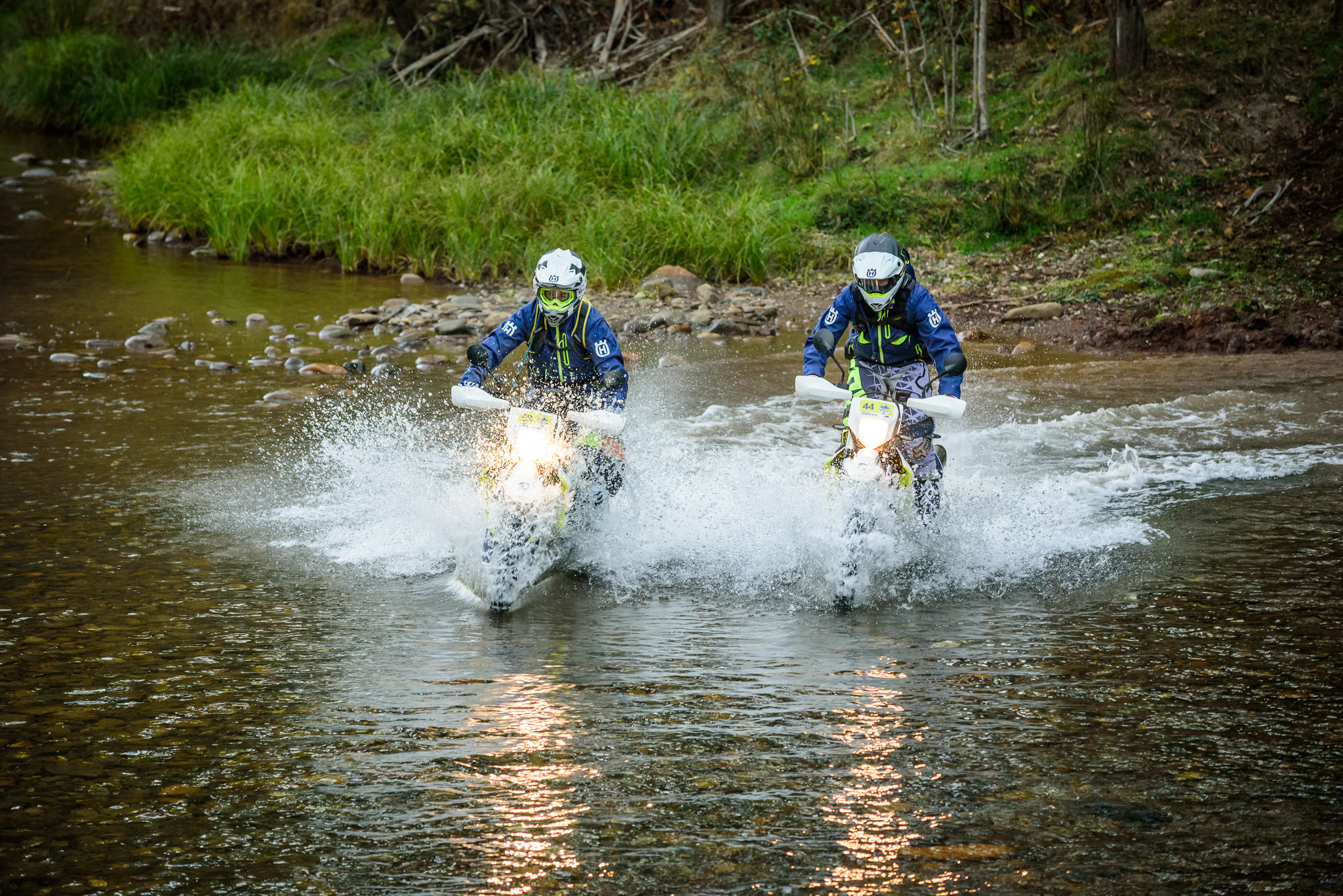In this dynamic photograph, two people are captured riding white dirt bikes at full speed through a shallow creek in a dense, dark forest. The riders, dressed in matching blue jackets and helmets that obscure their faces – one helmet an all-white design and the other a blue and white combination – power through the clear, almost translucent water, creating splashes and white froth all around them. The scene is illuminated by the headlights of their bikes, which cast bright reflections on the water's surface. Surrounding the creek, the bank is lined with tall green grasses, brown rocks, and gradually inclines into a hillside dense with trees and bushy areas. The entire setting exudes a raw, adventurous energy, accentuated by the natural forest backdrop and the palpable motion of the riders as they navigate the watery path toward the viewer.